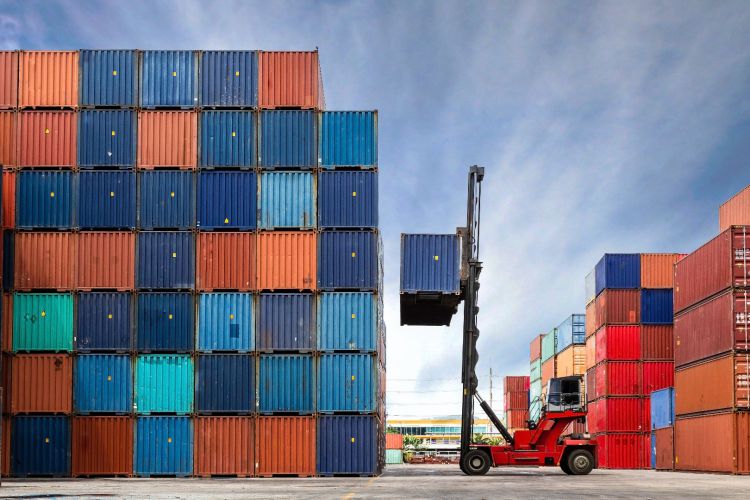The image captures a bustling shipping facility under a vivid blue sky scattered with feathery white clouds. The foreground prominently features a variety of colorful metal shipping containers stacked in rows, with vivid hues of blue, orange, green, and red creating a visually striking mosaic. To the left, the bottom row of containers alternates between blue and orange, with higher rows displaying a nuanced palette including dark blue, light blue, mid-tone blue, and greens. A central red-and-black crane is actively lifting a blue container, seemingly about to place it atop the existing stacks. On the right side, more containers are arranged in similar eclectic patterns, with notable sections featuring red and orange combinations. The facility extends into the background where a white and yellow building is partially visible. The ground is gray, marked with yellow lines, adding an industrial touch to the scene. The overall composition highlights the intricate and vibrant nature of container storage and handling operations.